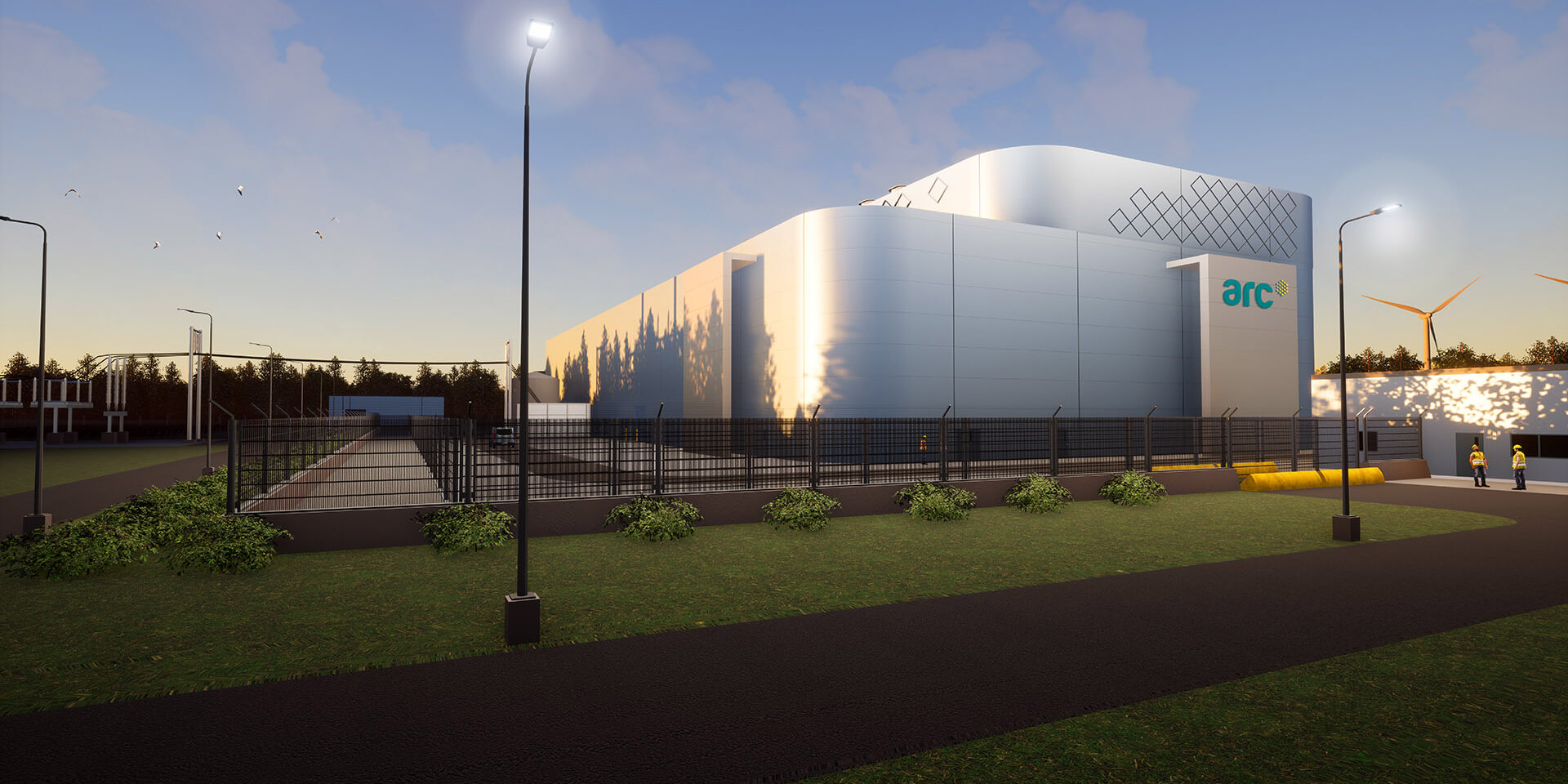The image depicts a detailed industrial or commercial building set in an outdoor scene that appears almost digitally rendered, reminiscent of an architect's concept or a CAD model. The large, multi-story silver building has a sleek, futuristic design with rounded corners, creating a softened, chrome-like appearance. On the front facade, the letters "ARC" in teal stand prominently alongside a latticework pattern visible near the top right corner.

Surrounding the building is a well-manicured landscape with an angular lawn and sporadically placed bushes. A wide, freshly paved walkway or driveway, about the width of two vehicles, extends around the building's perimeter, adorned with illuminated street lamps stationed regularly. These lamps cast light on the scene, suggesting either dusk or dawn.

Encircling the property is a chain-link security fence, possibly topped with barbed wire, enhancing the building's secured appearance. To the right side of the image are two workers in yellow safety vests and headgear, indicative of either hard hats or baseball caps, adding a touch of human activity to the scene.

In the background, two three-bladed wind turbines rise against a blue sky dotted with fluffy, white clouds, further hinting at the modern, eco-friendly nature of the facility. The scene is bathed in ambient daylight, with the sun casting reflective highlights on the building's silver surface.